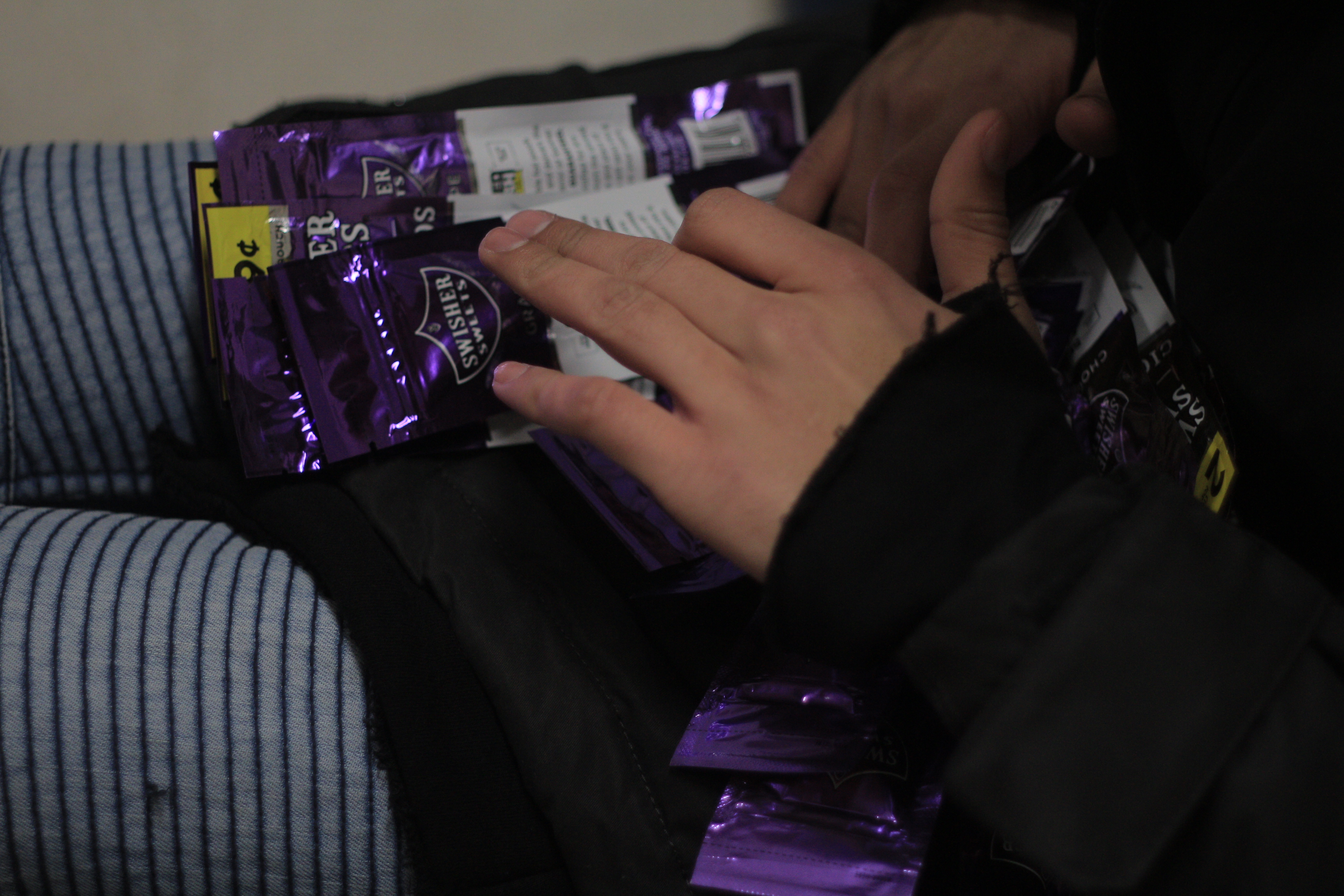The photograph captures a detailed scene centered around a pair of hands interacting with a collection of vertically arranged, narrow purple packets labeled "Swisher Sweets." The packets, displaying metallic purple and white accents, are adorned with white text and some yellow markings, including a scent icon. A Caucasian person is in the process of opening one of the packets, which sports a white nutrition facts label. This person's other hand is seen in the top right, possibly organizing the rest of the packets. The individual appears to be clad in light gray trousers with dark teal stripes. The setting is outdoors, evidenced by the natural lighting in the image.